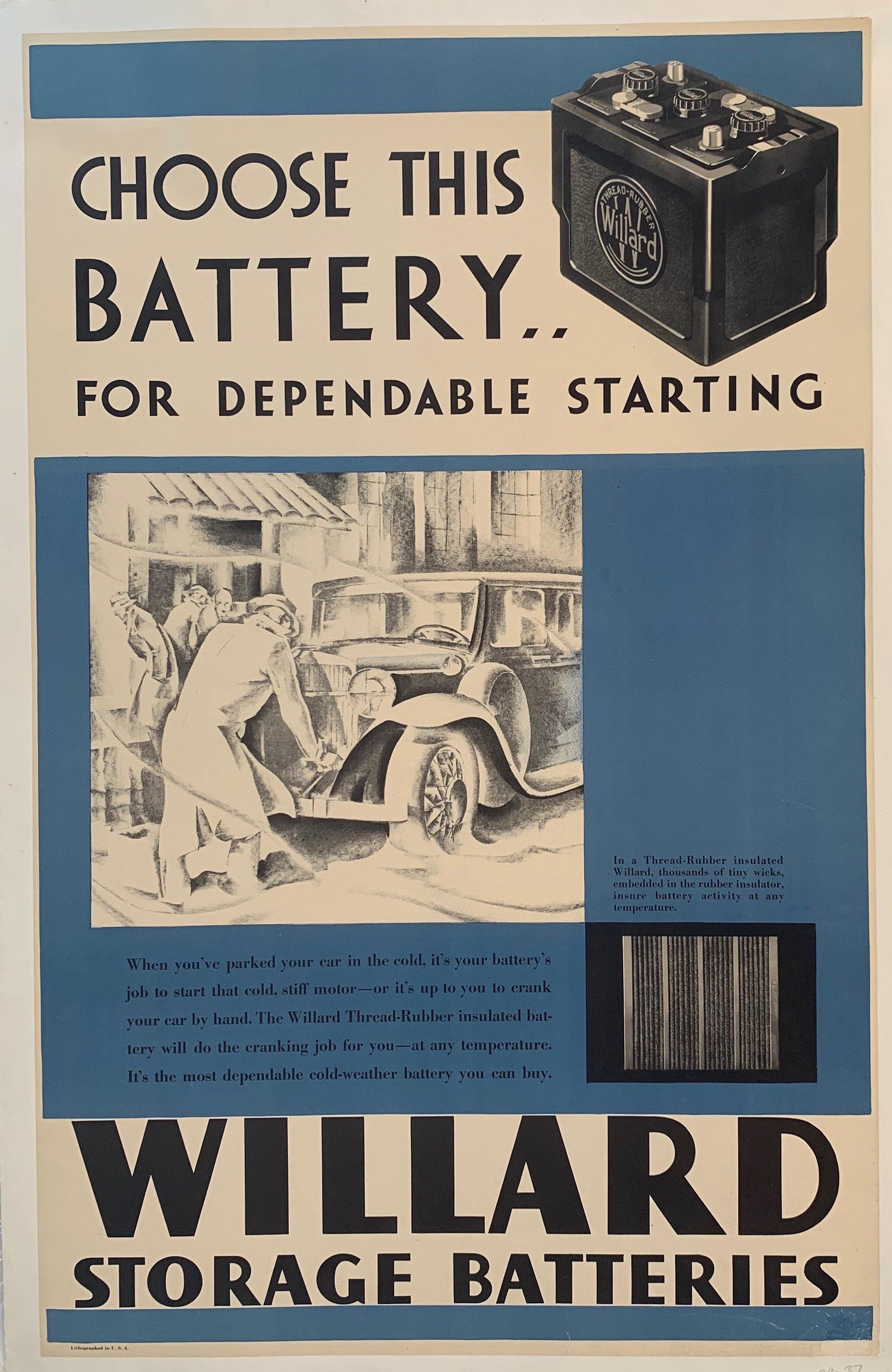The image depicts a tall, vintage advertisement banner with a worn-out, yellowed paper background and subtle blue highlights. Central to the advertisement is a black square Willard battery, illustrated in black and gray. The ad prominently features the phrase “Choose this battery for dependable starting” to the left of the battery illustration. Beneath this, there is a black-and-white drawing of a classic car, likely from the 1930s or 40s, with a man in a trench coat standing in front of the vehicle, possibly indicating a breakdown. The scene appears wintry, with white powder resembling snow on the ground. Towards the bottom of the ad, the text “Willard Storage Batteries” is boldly displayed. The banner also contains thin writing that is difficult to decipher and a small, indistinct image in the lower right corner.